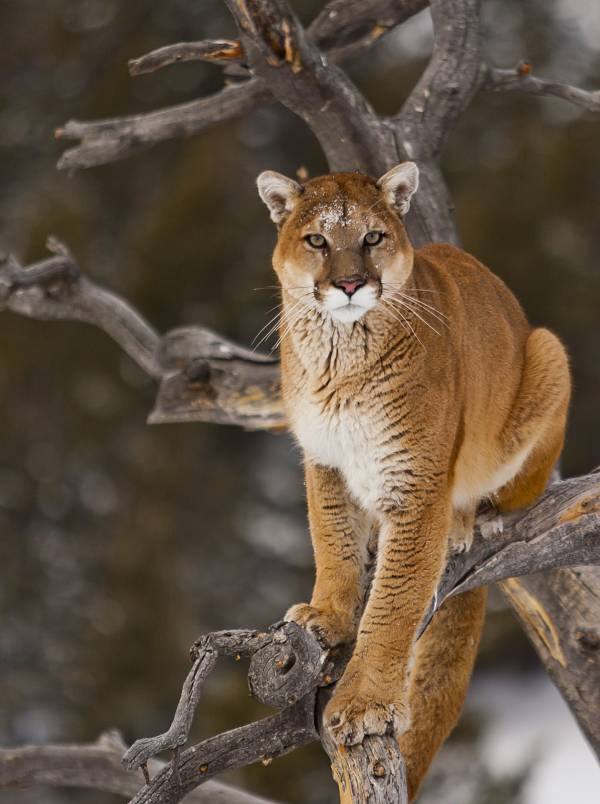This photograph captures a striking image of a mountain lion, also known as a cougar or puma, perched in a barren tree devoid of leaves, suggesting a winter setting. The cougar, a large light brown feline with rusty brass undertones, has patches of lighter, almost white fur on its muzzle, chest, and stomach. A hint of snow adorns its forehead. It gazes intently at the camera, slightly off to the viewer's right, with its reddish nose and prominently large paws visible. The feline appears half-sitting, with its front body erect as if it has just noticed something, giving a sense of attentive alertness. The background is heavily blurred, emphasizing the cougar and lending a mysterious, forest-like backdrop to the scene.